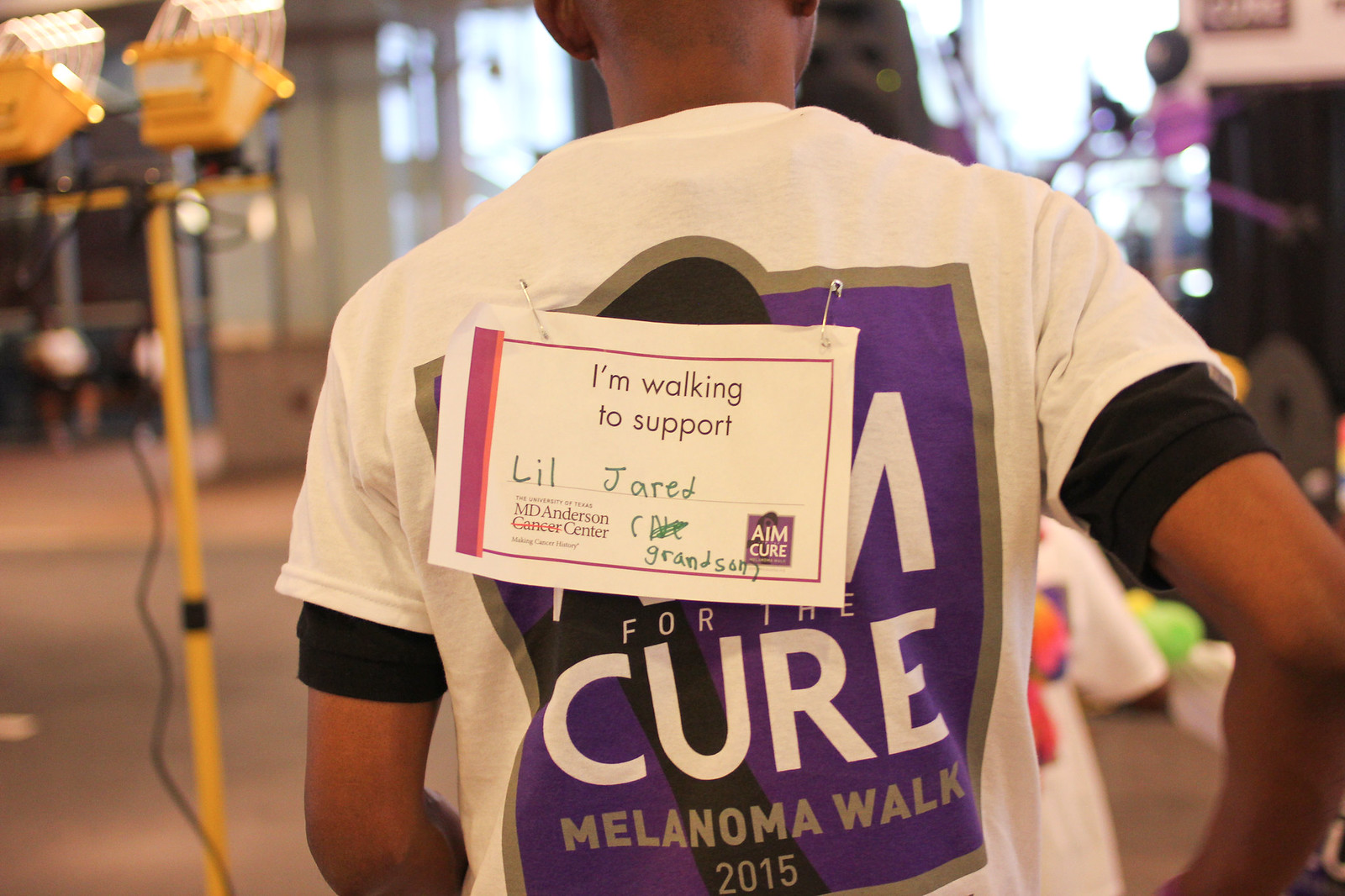This full-color nighttime photograph from 2015 captures a moment during the Melanoma Walk. A man with somewhat dark skin is in focus, seen from behind, walking forward. He wears a blue t-shirt over a black undershirt. Safety-pinned to his shirt is a sign that reads, "I’m walking to support Lil' Jared. Aim for a cure. MD Anderson Cancer Center." 

The scene is illuminated by yellow spotlights, and the surroundings include lit-up building windows and doors, suggesting an urban environment. Additional tall yellow pipes are visible, adding to the industrial feel. In front of the man, there is a little kid, either just finishing the walk or preparing for it. Overall, the image encapsulates a moment of solidarity and hope in the fight against melanoma.